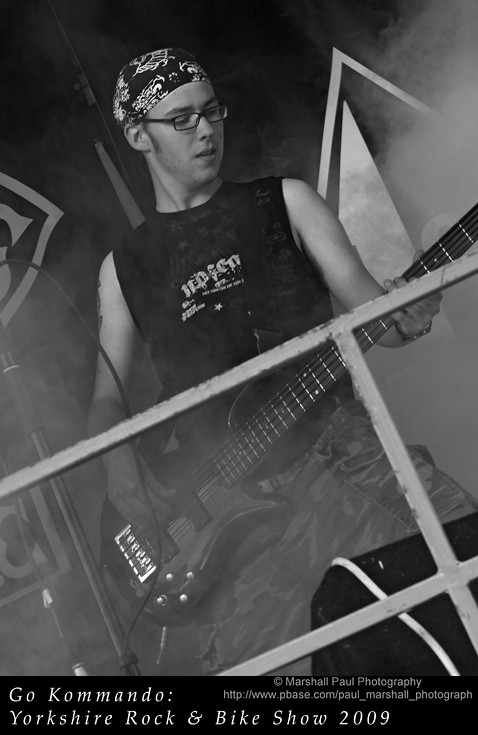The image is a tall, black and white photograph centered on a Caucasian male guitarist captured from the knees up. The man is standing in the middle of the frame, holding an electric guitar at his left hip while strumming with his right hand. He is dressed in camouflage cargo pants and a sleeveless black shirt with white lettering, possibly reading "no fear." His light skin is adorned with visible tattoos on his upper arms. He wears rectangular glasses and a black and white bandana on his head. In the background, smoke creates an atmospheric effect, suggesting he is performing live on stage. A metal fence or gate runs diagonally in front of him, enhancing the stage feel. At the bottom of the image, a black rectangle features italicized white text that reads, "Go Commando, Yorkshire Rock and Bike Show 2009," accompanied by the smaller text, "Marshall Paul Photography." The image suggests a dynamic concert setting, with additional equipment like a speaker or amplifier and possibly a microphone in the vicinity.